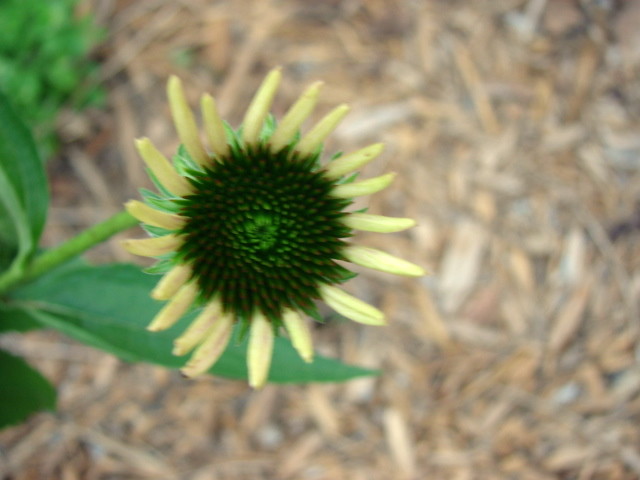A close-up image of a sunflower that has just barely opened. The central bloom is surrounded by dark green or black spikes, transitioning to vibrant lime-green petals arranged in a circular pattern reminiscent of a sunflower. Outside the green petals, there's a layer of pale yellow spikes that curve upward and around, almost resembling the rays of the sun. The flower is attached to a green stem that extends downward and to the left. A large green leaf, partially obscured by the flower, stretches from the left side toward the center. Another leaf is visible on the left, extending upward and out of the frame. The background is very blurred, with hints of brownish wood chips or dead grass, and patches of green foliage, creating a soft, muted backdrop that emphasizes the flower’s vibrant colors.